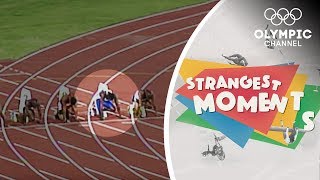The image is divided into two distinct parts, with the left side featuring a track and field event and the right side displaying branded content. On the left, four runners are at the starting line of a red track, poised to begin their race. The third runner from the left is highlighted, suggesting they are of particular interest. The background includes visible sections of grass, indicating the event takes place in an outdoor field setting. 

The right side of the image displays the text "Strangest Moments," with an abstract pattern of straight lines in red, green, blue, and yellow behind it. At the top, the five Olympic rings are prominently displayed above the text "Olympic Channel," indicating that this is a segment from a show on the Olympic Channel that focuses on unusual or notable events in Olympic history. The overall composition of the image suggests that it highlights one of the peculiar moments captured during the Olympics.